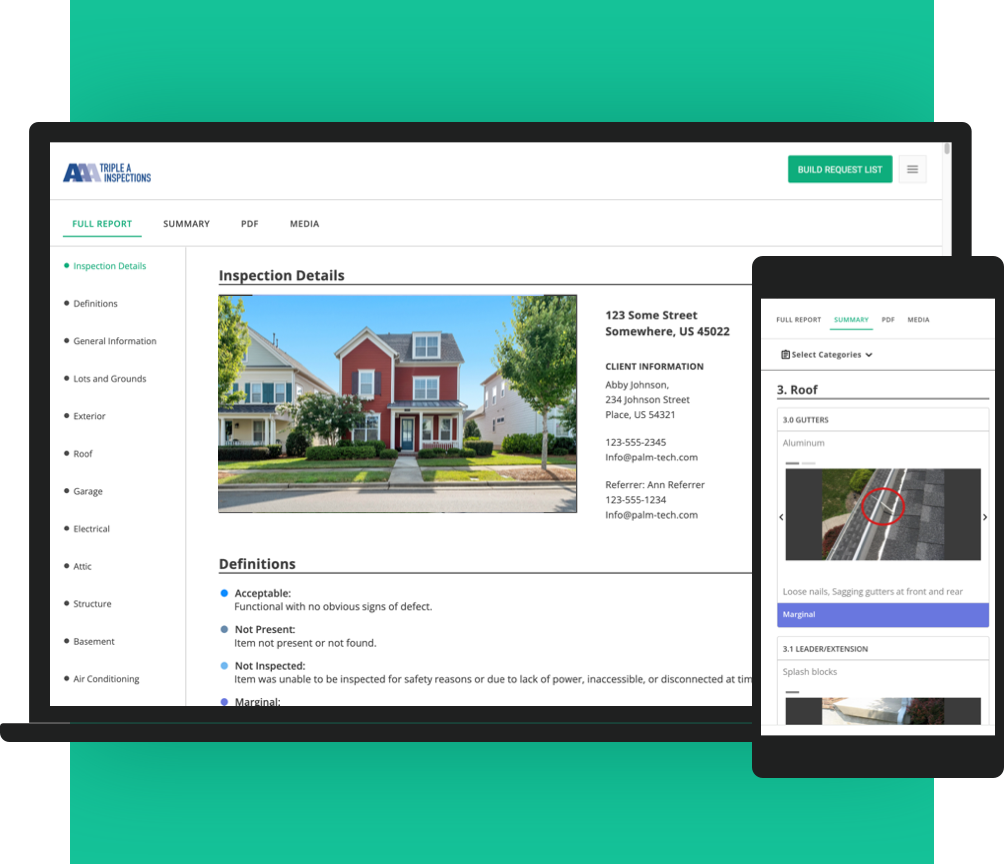The screen displays a comprehensive inspection report from AAA Inspections. On the left side, the "Full Report" tab is highlighted in green, with options for "Summary," "PDF," and "Media" beside it. Below these options, "Inspection Details" is also highlighted in green. The report provides various pieces of information, including an address—123 Soma Street, Somewhere, USA, 45022—and client information: Abby Johnson, residing at 234 Johnson Street, Place, USA, 54321, with the contact number 123-555-2345. It also lists an email contact, Refer, Anna Refer, along with the number 123-555-1234. Definitions for terms such as "Acceptable," "Not Present," and "Not Inspected" are included, and to the right, the "Summary" tab is highlighted in green. The summary section displays details about the roof, specifying it as aluminum, along with a picture of the roof shown in a smaller screen with a green background.